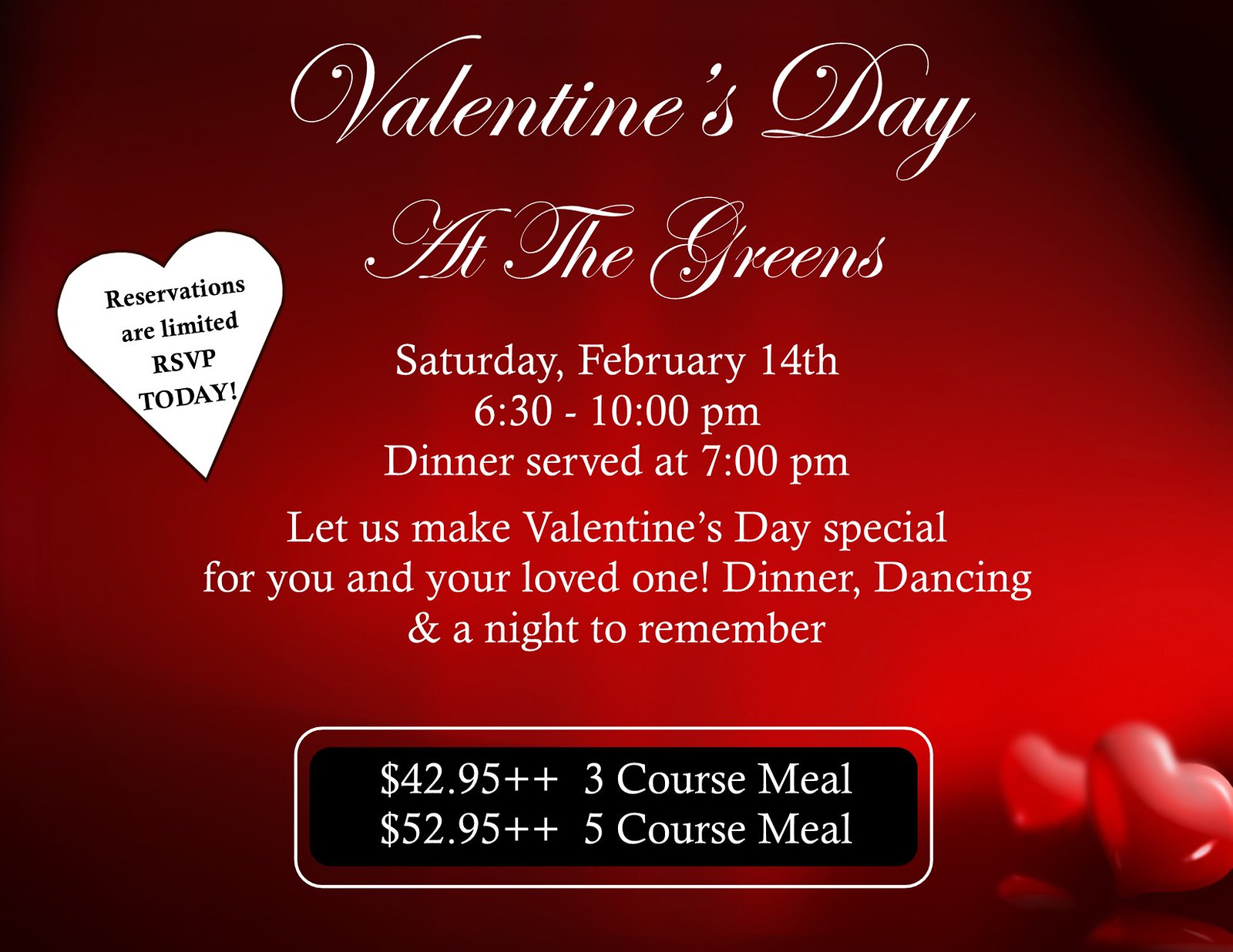The image is an invitation card for a Valentine's Day event titled "Valentine's Day at the Greens" in an elegant, cursive font at the top. The background is predominantly burgundy red with a lighter red gradient in the center and black edges at the four corners. In the top left-hand corner, a white heart contains the text "Reservations are limited, RSVP today" in black font. Below the title, the event details are written in white font: "Saturday, February 14th, 6:30 to 10 p.m. Dinner served at 7 p.m." The invitation promises to make Valentine's Day special with "Dinner, dancing, and a night to remember." At the bottom of the card, a black rectangular box with a white outline offers two pricing options in white letters: "$42.95++ for a three-course meal and $52.95++ for a five-course meal." The bottom right corner features two shiny red hearts that reflect off the edges.